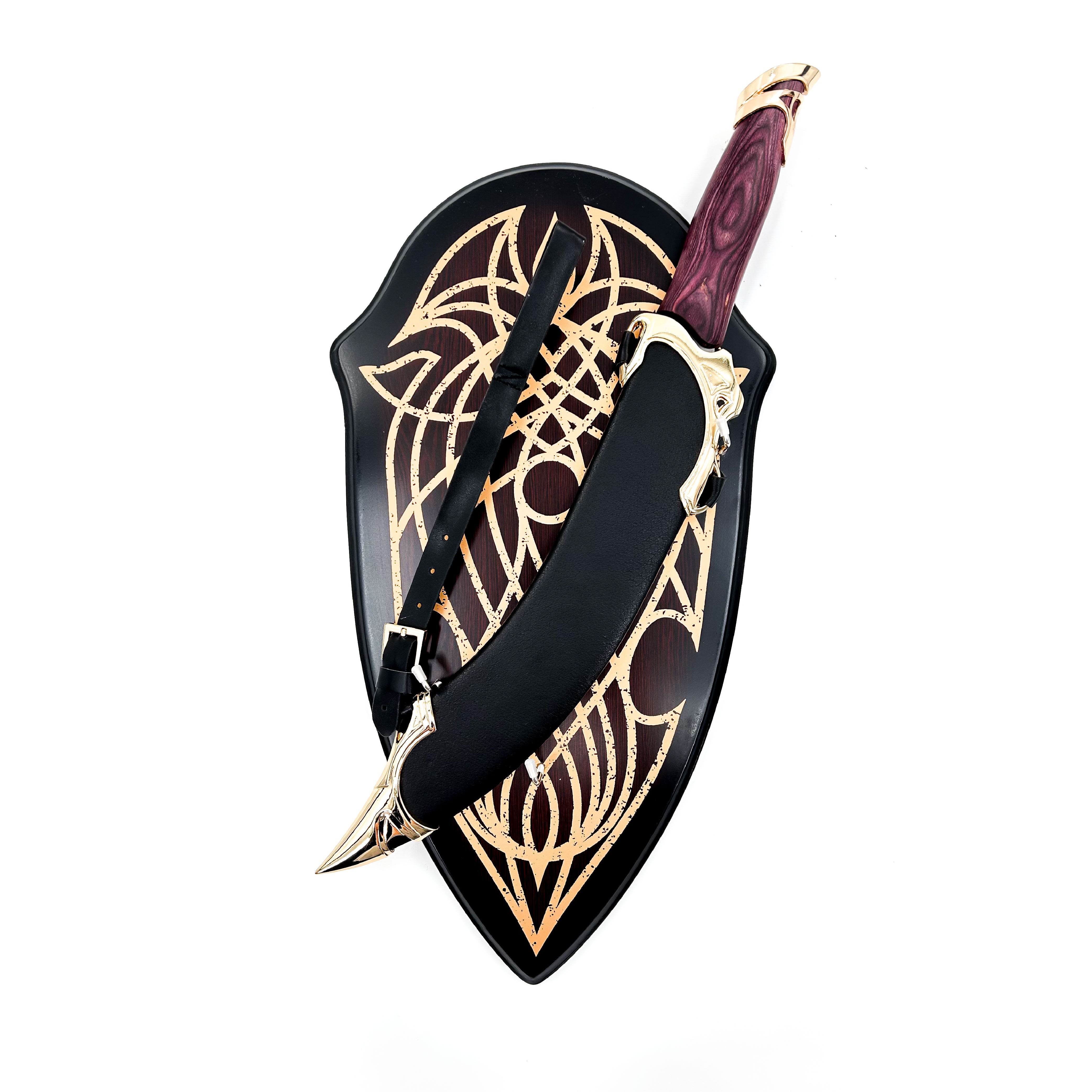This product photo showcases an ornamental sword sheathed in a leather scabbard adorned with gold or brass decorations, suspended by a strap. The handle of the sword, which resembles a decorative kukri or scimitar, is crafted from mahogany-esque wood. The sword is positioned over a wooden shield that complements the sword's handle in tone. The shield features a burnt edge that darkens around its perimeter and includes intricate, possibly Celtic or elvish, inlaid lighter designs. The overall aesthetic exudes a medieval or Middle Eastern vibe, while the front-facing arrangement and stark white background suggest that the photo is intended for an e-commerce setting, emphasizing the detailed craftsmanship and decorative appeal of the set.